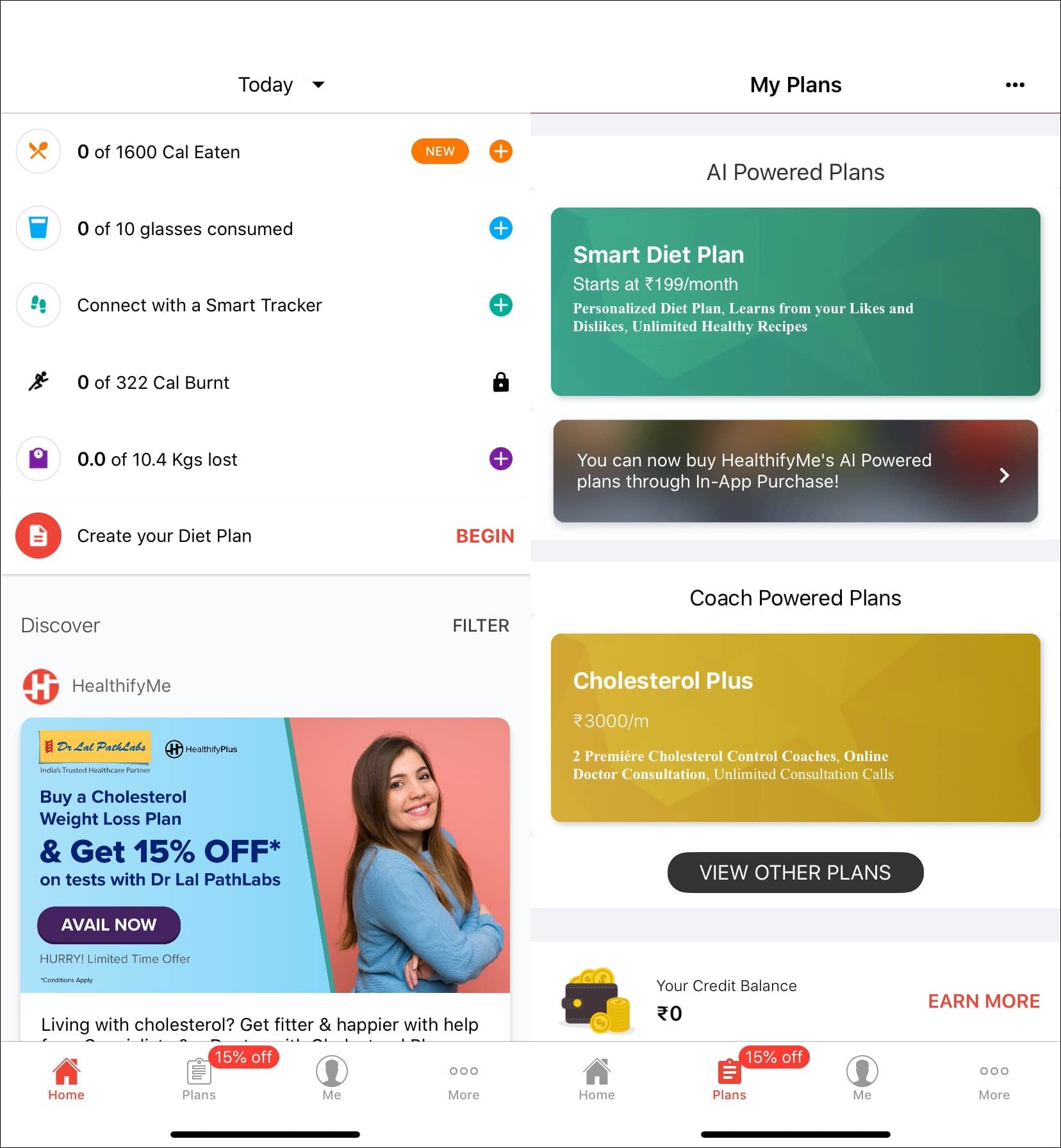A screen capture of an online application page with a clean white background. The header section, on the left, prominently features the word "TODAY" in black, accompanied by a drop-down arrow to its right. On the upper right side of the page, the phrase "MY PLANS" is clearly visible. Directly below "TODAY," detailed metrics are displayed, including calories consumed, glasses of water drunk, and a connection status with a smart tracker. A striking image of a smiling woman in a blue top, highlighted in blue and pink, is positioned below the metrics. To the left of the woman, a bold blue callout reads "AND GET 15% OFF." On the right side of the image, there are three rectangular frames with rounded corners: the top frame has a green background, the middle frame is grey with red accents, and the bottom frame is a rich golden yellow.